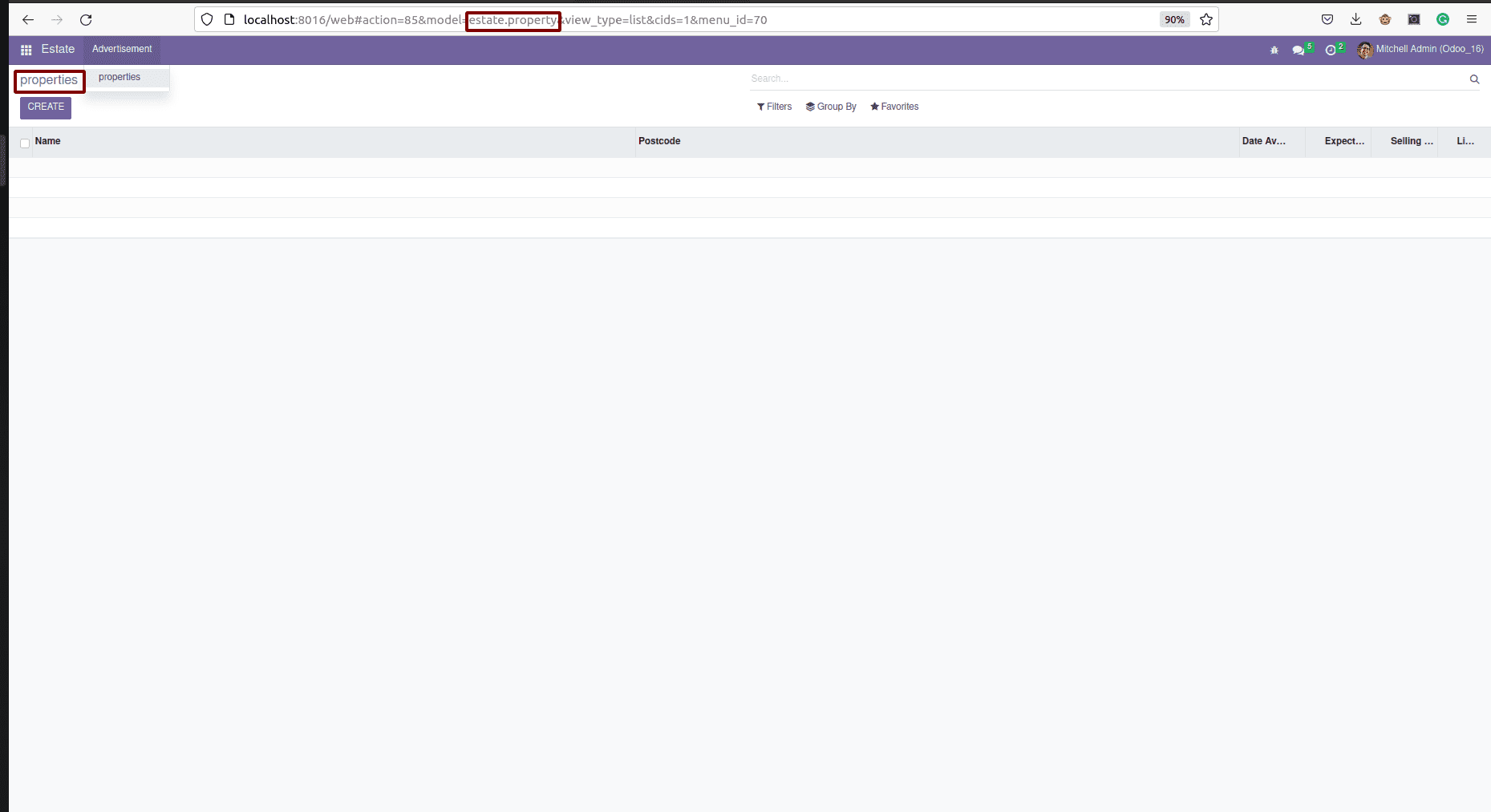The image displays a web page with a predominantly white background, accentuated by various elements in red, purple, green, and black. At the very top of the page, navigation buttons such as a back arrow, a refresh arrow, and a shield icon in the web bar indicate its local host nature. A red box highlights the text "estate property," drawing attention to this section. Additional interactive features include a star icon for favoriting the page and both green and red buttons, presumably for different actions. The header bar, colored in purple, reads "Estate Assessment is Next" and includes several white buttons containing green boxes, as well as a profile button. Below the header, the term "properties" is outlined in red on the white background. A prominent purple "create" button stands out among the options available.